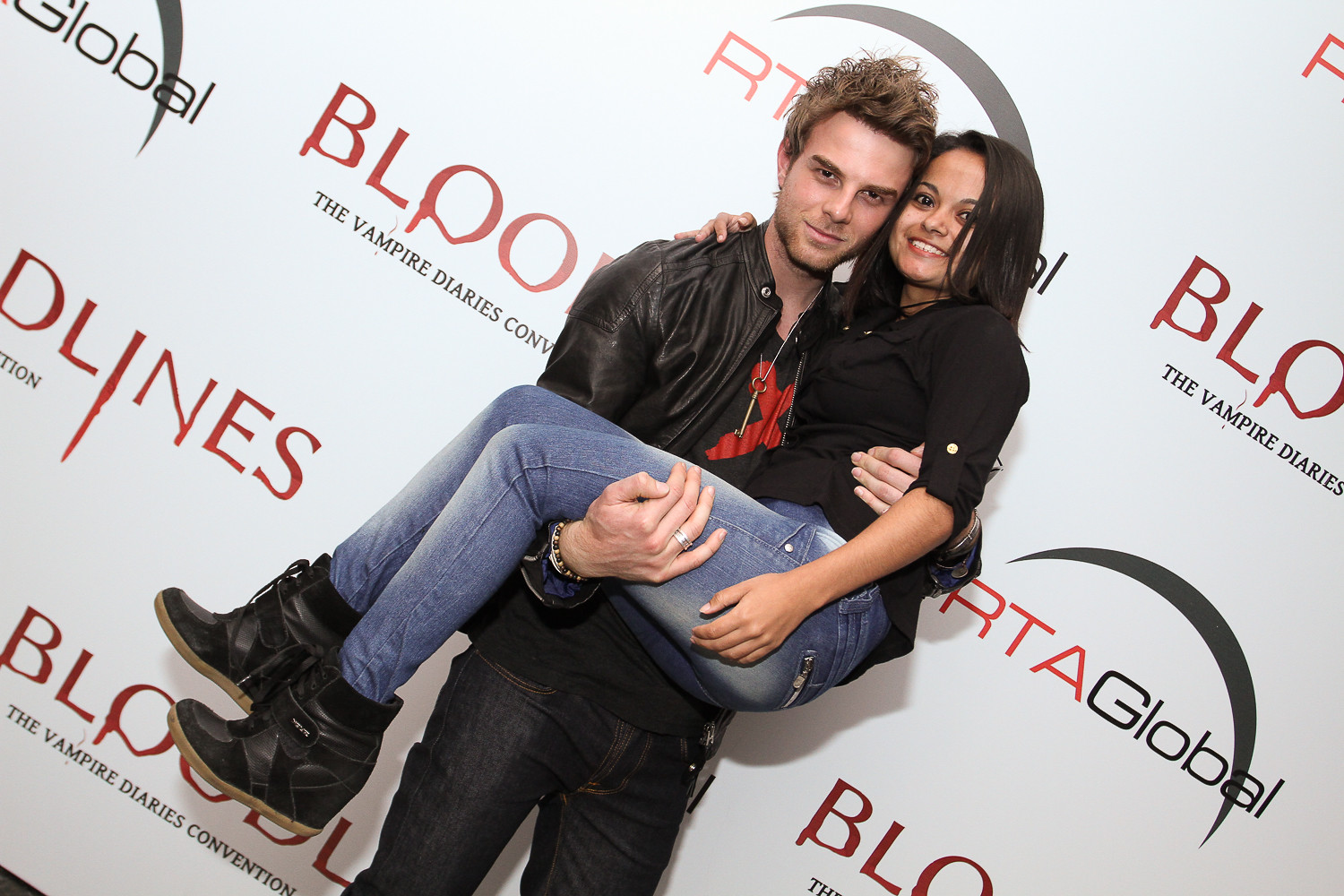In this color photograph with a slight rightward tilt, two individuals are prominently featured against a promotional backdrop for "The Vampire Diaries: Bloodlines." The man, identified as Bjorn Haras, sports short, spiky, blonde-tipped hair and is dressed in a black leather jacket, black shirt, and black pants. He is carrying a young woman, who is dressed in a black top, blue jeans, and black boots, by the legs. Both individuals are smiling directly at the camera. The backdrop showcases multiple instances of the "Bloodlines" logo, complete with red blood-like drips on the zeros, and includes the "The Vampire Diaries Convention" text in small black letters below. Additionally, the logo of RTA Global, characterized by red lettering and the outline of a circle, is visible on the white banner. The attire of the pair, while dark and casual, stands in contrast to the typical red carpet fashion, suggesting either an informal promotional event or a candid moment with a fan. The photograph is captured in a style that emphasizes realism and representational detail.